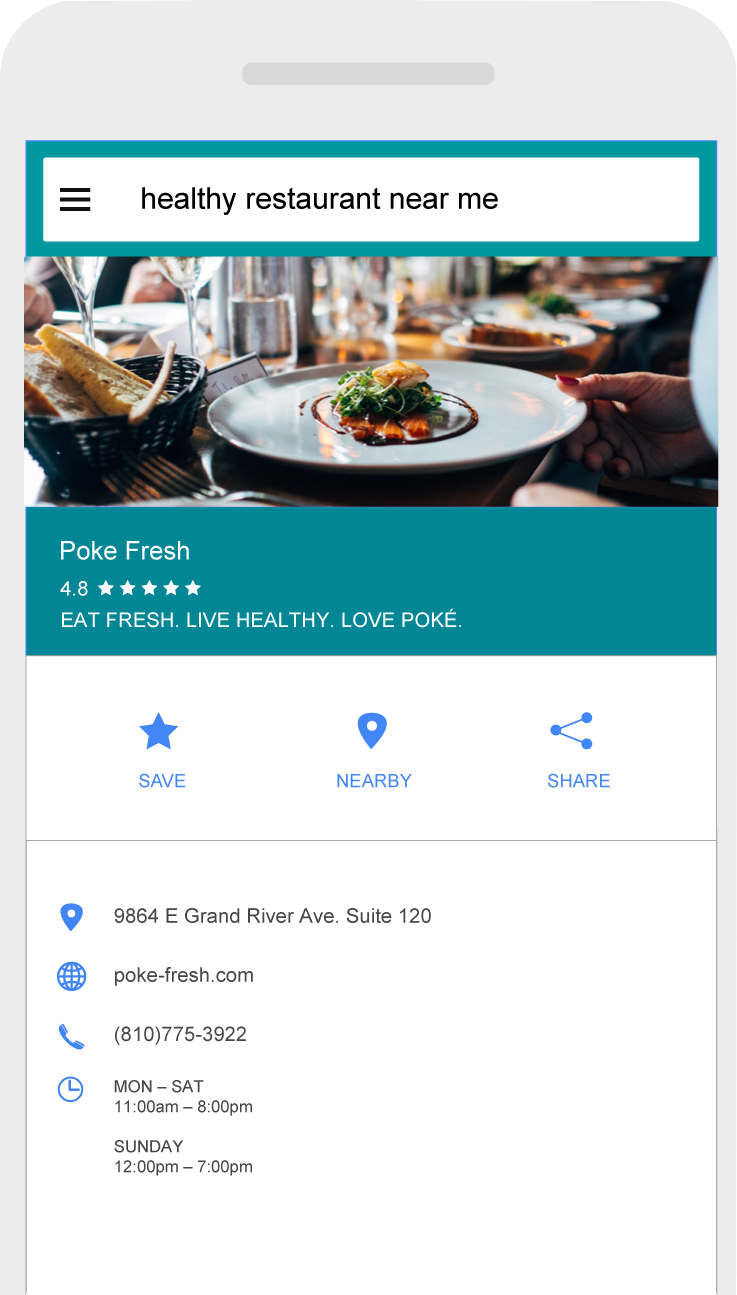The image depicts a cell phone screen displaying a restaurant listing. At the top, a gray border, which is part of the phone itself, is visible. Below this, a white rectangular banner with a thick blue border houses the text "Healthy Restaurant Near Me," accompanied by three horizontal lines stacked vertically on the left side. 

Directly below the banner, a photograph captures the inside of a restaurant. The primary focus is a plate of food being touched by a person's hand. In the background, another table is visible, adorned with glasses and additional plates of food, suggesting an inviting dining atmosphere. 

Beneath the photograph, text reads: "Poké Fresh 4.8 stars. Eat fresh, live healthy, love Poké." Following this description, there is a row of interactive icons:

1. A blue star icon labeled "SAVE,"
2. A pin icon labeled "NEARBY" in blue text,
3. An interconnected dots icon labeled "SHARE" in blue text.

Further down, additional details about the restaurant are provided. A pin icon followed by the address reads: "9864 East Grand River Avenue, Suite 120." Next to a globe icon, the text "pokefresh.com" is displayed, and beside a phone icon, a contact number is listed. Finally, an image of a clock provides the operating hours: "Monday through Saturday 11 a.m. to 8 p.m., Sunday 12 p.m. to 7 p.m."